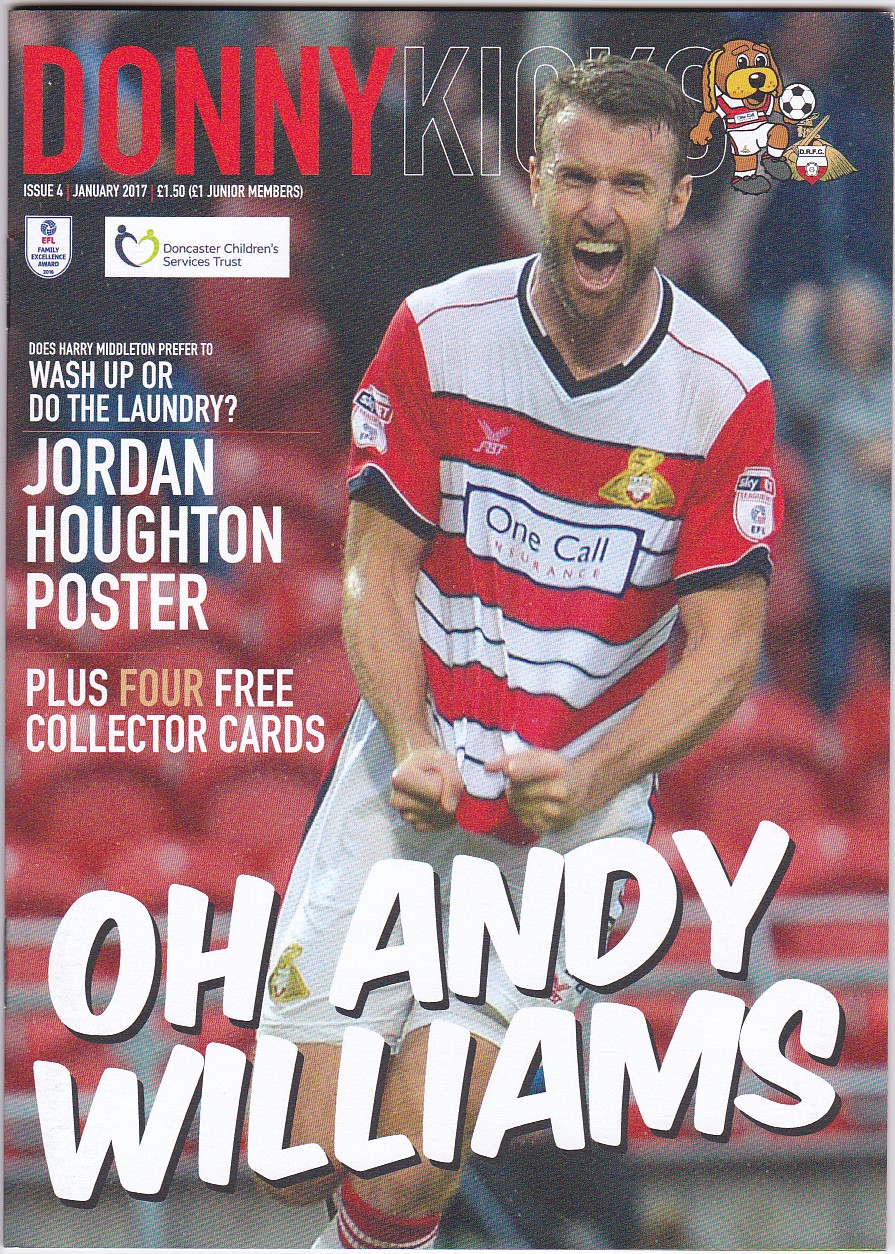This is the cover of a soccer magazine titled "Donnie Kicks," as indicated by the partially obscured title at the top. Featured predominantly on the cover is a celebratory soccer player with short brown hair and light skin, wearing a white, red, and blue top, white shorts, and red and white striped socks. He is clenching his fists, his mouth open in a joyous yell, suggesting he has just scored a goal or won a game. Below him, in all capital white letters, it states, "Oh, Andy Williams," identifying the player. 

Above Andy Williams, there's a cartoon of a dog kicking a soccer ball, adding a playful touch to the cover. 

To the left of the player, the issue is marked as January 2017, and the price is listed as £1.50, or £1 for junior members. Additional text on the left reads, "Does Harry Middleton prefer to wash up or do the laundry?" followed by "Jordan Houghton poster" and "plus four free collector cards," with the word 'four' highlighted in yellow.